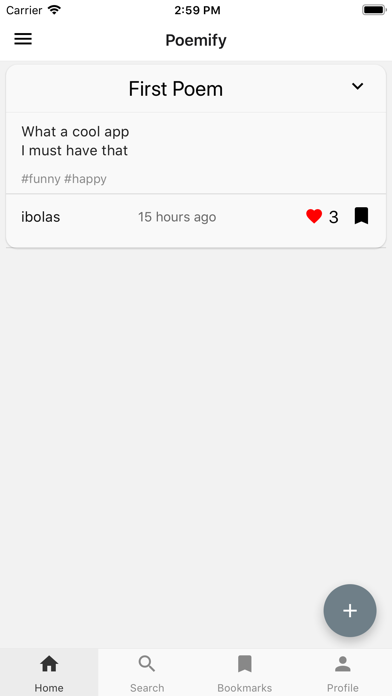A phone screenshot taken at 2:59 p.m. with full carrier bars and a fully charged battery. The screen displays an app titled "Poemify." The main feature of the screen is the first poem, which is accompanied by a drop-down context menu on the right-hand side. The bottom left corner showcases a three-lined context menu. The bottom right has a gray plus icon, presumably for adding content. The bottom of the screen includes navigation icons: a house for Home, a magnifying glass for Search, a tapestry flag for Bookmarks, and a person icon for Profile. The caption notes that "Poemify" appears to be an intriguing app, with hashtags #funny and #happy provided by the user iBolas, 15 years ago. There are no additional notable elements in the screenshot.